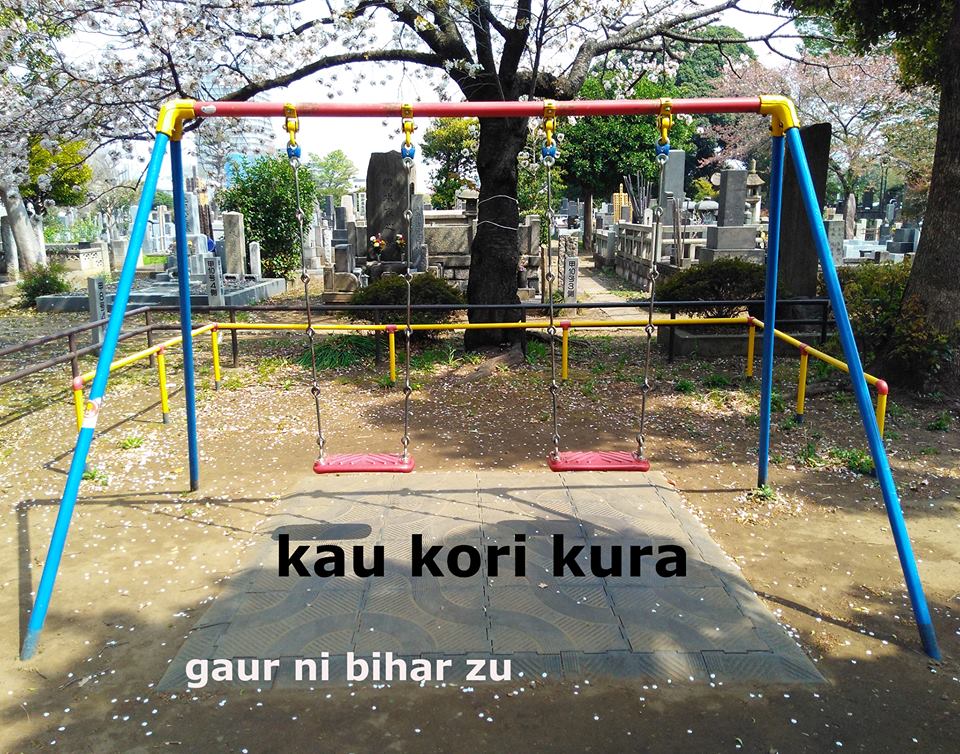The image features a vibrant swing set with metal bars prominently in the foreground. The swing set includes two red seats hanging from sturdy metal chains. The frame of the swing set is a combination of blue and red with touches of yellow, adding a cheerful pop of color amidst the surroundings. Underneath the swings, the ground appears to be either concrete or a dense plastic, while the surrounding area is primarily dirt. In the background, a cemetery is visible, featuring numerous headstones, which exhibit characteristics suggesting an Eastern, possibly Japanese, origin. A large, captivating cherry blossom tree, along with green trees, enhances the scenic backdrop. A small yellow fence separates the playground from the cemetery. Text at the bottom of the image reads "Kao Kore Kura" in black, with "Gaori Bihar Zoo" in smaller white text below it.